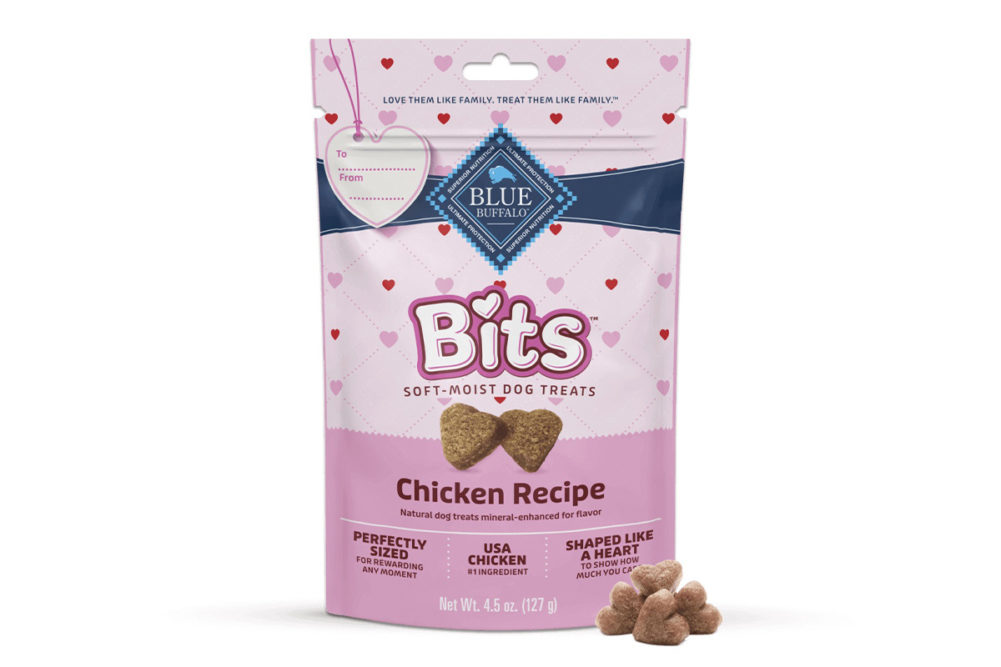This image showcases a bag of dog treats from Blue Buffalo Brand, specifically their Bits Soft Moist Dog Treats in a chicken recipe flavor. The bag is designed to be cutesy and festive, featuring a primarily light pink color with a pattern of pink and red hearts. The top three-quarters of the pouch displays a diamond-like grid with small hearts at the intersection points, while the bottom quarter is a darker pink bearing essential information such as "perfectly sized USA chicken" and the net weight of 4.5 ounces. The bag includes both Blue Buffalo's distinctive diamond-shaped logo at the top, surrounded by a ribbon design, and another prominent pink-outlined white logo for Bits. The bag is resealable with a tear top and has a "To From" label imprinted as a Valentine’s gift feature along with the text "Love them like family, treat them like family" in tiny print. On the front of the bag, an illustration depicts the heart-shaped treats, and four of these treats are showcased outside the bag for added detail.